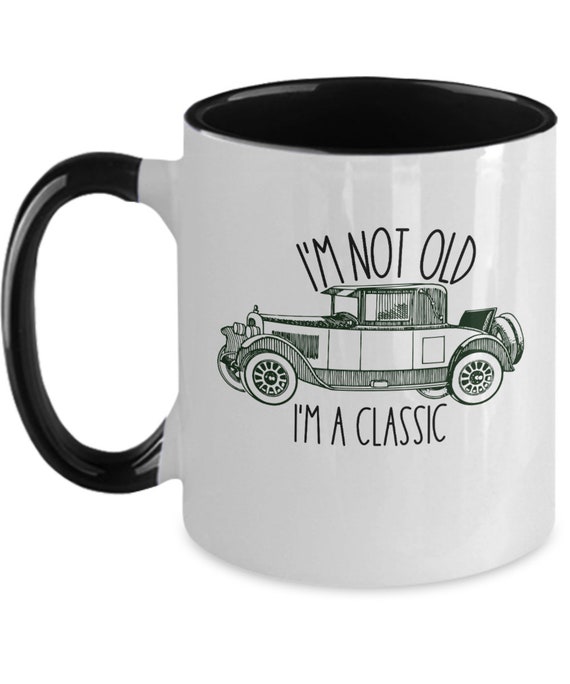This image showcases a stylish coffee mug with a glossy white exterior and a glossy black interior. The mug features a sleek, black handle, which is partially white at the top and bottom. The design on the front of the mug displays an illustration of a classic car from the 1920s or 1930s, complete with spoked wheels, a spare tire on the back, rounded fenders, and a low-profile canopy cab. The body of the car is segmented by black lines, with vertical dark lines shading the lower portion. Above the car, tall, thin black letters read, "I'M NOT OLD," and below the car, it continues, "I'M A CLASSIC." This evocative design, combined with the shiny black and white color scheme, makes the mug not only functional but also a nostalgic piece of art.